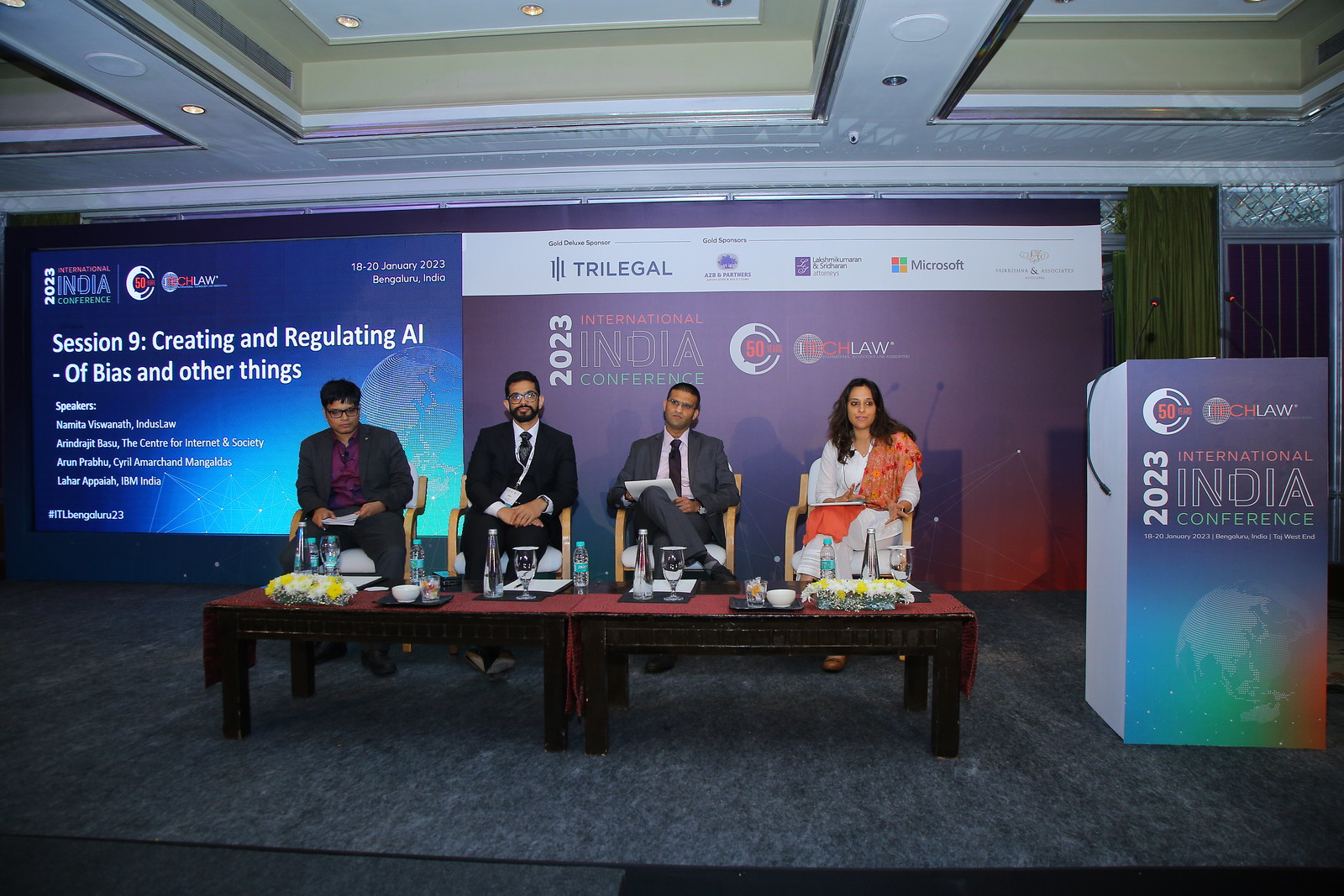The photograph depicts a panel discussion at the 2023 International India Conference. The stage features four panelists seated in wooden chairs behind two dark coffee tables adorned with drinks and food. From left to right, the panelists include three men and one woman, all appearing to be of Indian descent. The man on the far left is dressed in a violet shirt paired with business attire, while the two men in the center are wearing business suits, one with a tie and one without. The woman on the far right stands out in a white dress with an orange sash. A lectern positioned to the right of the panelists bears the conference name, and behind them, large posters and screens display the session title: "Session 9: Creating and Regulating AI of Bias and Other Things," along with various logos, including Microsoft. This setup clearly indicates that the ongoing discussion is focused on AI topics.